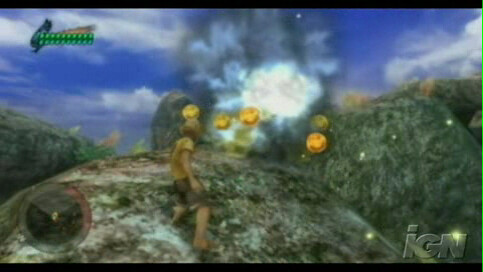The image is a blurry screenshot from a video game, displayed on a television screen. The gameplay scene is set outdoors during the daytime with a bright blue sky dotted with white clouds. The central figure is a young Caucasian male character, dressed in brown shorts and a yellow short-sleeved shirt, who is positioned atop one of three stone mountains. Surrounding him are small, yellow smiley faces or gold globes that float in the air. There is a notable feature of a small explosion nearby, with a white cloud of smoke illuminated by gray hues. The screen also includes various on-screen elements: in the lower right corner are the letters "IGN," with the "I" in lowercase and the "G" and "N" in uppercase. The top and bottom of the image have black borders, and the lower left corner contains two concentric circles with a dot in the middle, likely serving as a compass or game indicator. Additionally, in the upper left corner, there is a partially visible green word or icon, which may represent the player's status or power level.